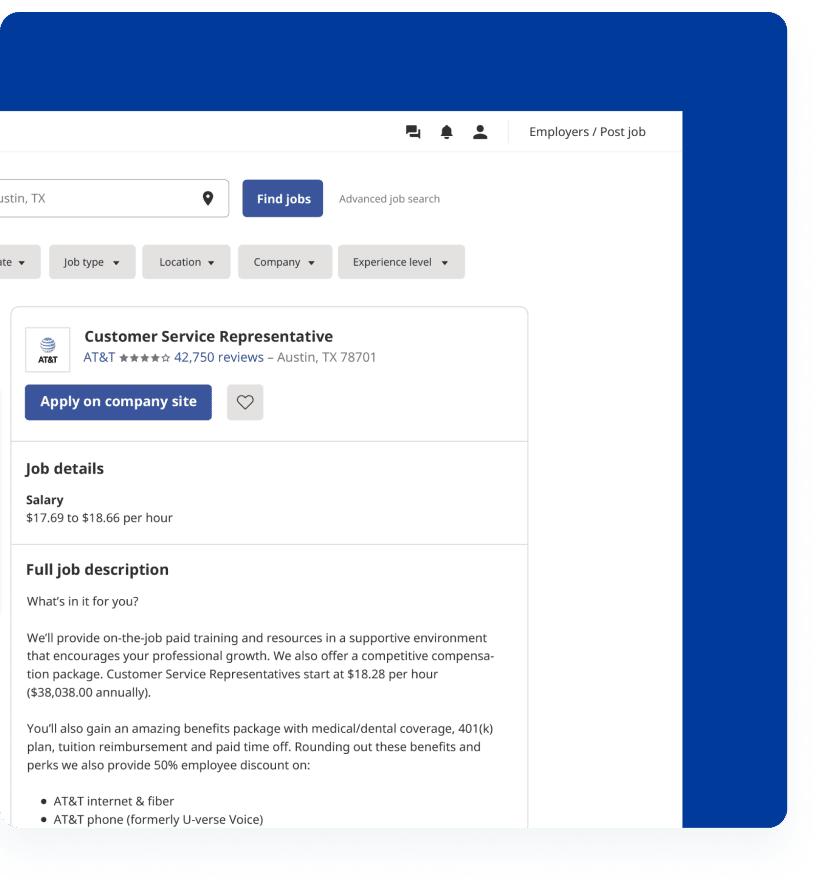**Detailed Job Listing Screenshot Description:**

The image displays a screenshot of a job listing with a blue border encasing a white background webpage. The job location is specified as Austin, TX (Texas) with the postal code 78701. Prominent on the page is a "Find Jobs" button in blue, along with an "Advanced Job Search" option.

Filters are available for sorting job listings by job type, location, company, and experience level. The highlighted listing is for the position of Customer Service Representative at AT&T. The company's logo, a blue globe symbol followed by the letters "AT&T" in black text, is prominently displayed. A star rating of 4 out of 5, based on 42,750 reviews, is shown in gray.

Further details include a button to apply on the company site and a heart icon, likely for saving the job listing. The job details section specifies that the salary range is from $17.69 to $18.66 per hour. It also includes a detailed job description highlighting the benefits and compensation package:

- Starting hourly wage is $18.28, with an annual salary of approximately $38,038.
- The job offers a comprehensive benefits package including medical and dental coverage, a 401(k) plan, tuition reimbursement, and paid time off.
- Additional perks include a 50% employee discount on AT&T internet and fiber services, as well as AT&T phone services (formerly known as U-verse Voice).

The description conveys a supportive working environment with on-the-job training and resources to encourage professional growth.